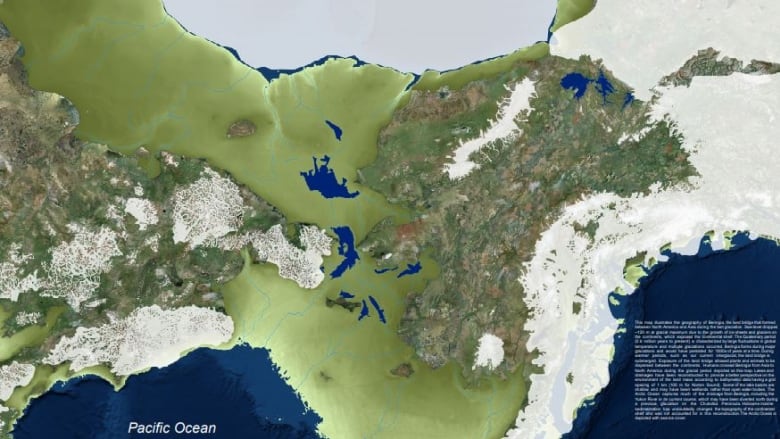The image appears to be a detailed, computer-generated topographical map displaying varying geographical features with depth and dimension. On the bottom left corner, there is a clear label for the Pacific Ocean, while a large green landmass extends across the map, interspersed with patches of white that likely indicate snow-covered areas. The terrain within this green expanse shows depth through different shades of green and brown, suggesting the presence of hills and mountains, particularly visible on the right-hand side. Small blue sections scattered throughout the map represent bodies of water, such as lakes. The top part of the map is predominantly white, hinting at snowy regions. The bottom right corner contains a passage of text that is too blurred to read, further suggesting the image might be part of a book or a document. This map does not pinpoint specific locations but rather illustrates the general geography and varied topography of the land depicted.